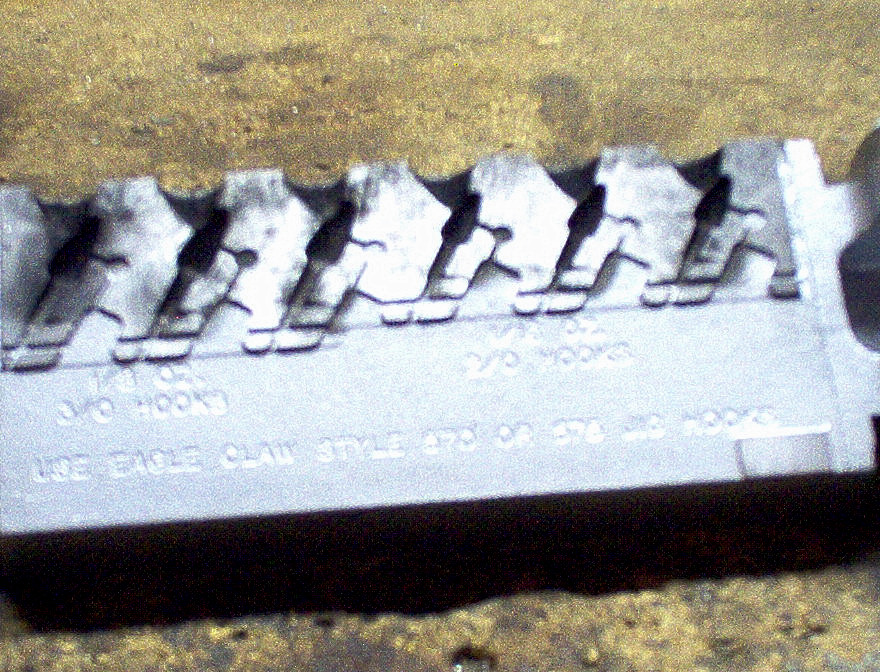This is a blurry close-up image of a rectangular piece of metal, likely a tool, laying on what appears to be a brownish stone or possibly oil-stained granite surface. The metal object features a series of teeth along the top edge, diagonally arranged, with around seven teeth visible, though some are almost completely washed out by light reflection. Engraved on the metal are the words "U05 Eagle Claw style" along with a series of numbers, though parts of the text, including the word "hooks," are somewhat obscured by the reflection. The bottom of the metal piece runs horizontally across the middle of the image, and the right edge shows two extensions protruding out of the frame.